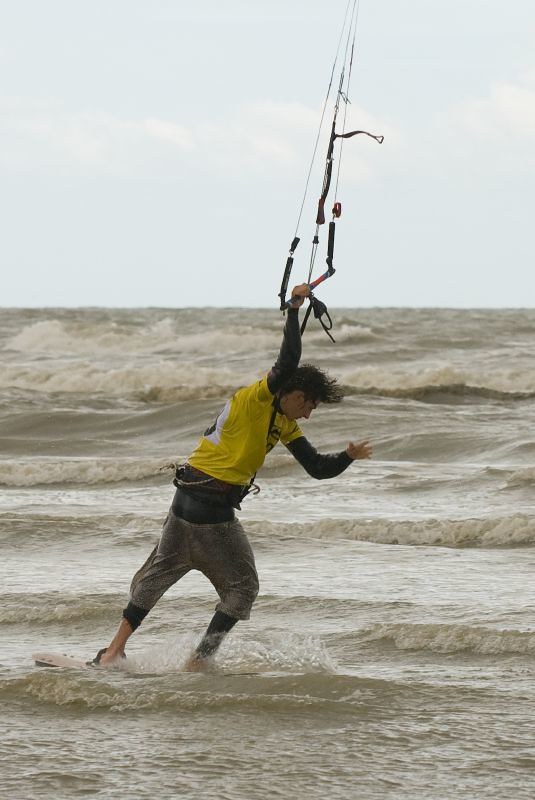The image depicts a young man engaged in a water sport, possibly windsurfing or kiteboarding, on a choppy, murky green ocean under a hazy gray sky. His messy, dark hair is wet, and he's wearing layered clothing that includes a yellow t-shirt over what appears to be a wetsuit, and gray pants that stop above his ankles. The man is balanced on a thin board with his feet strapped in, leaning precariously to the right. His right hand grips a hang glider bar connected by wires to a parachute kite that's out of frame. He extends his left arm forward in an attempt to maintain his balance amid the rough waves. The overall scene reflects a dynamic and challenging moment on the water.